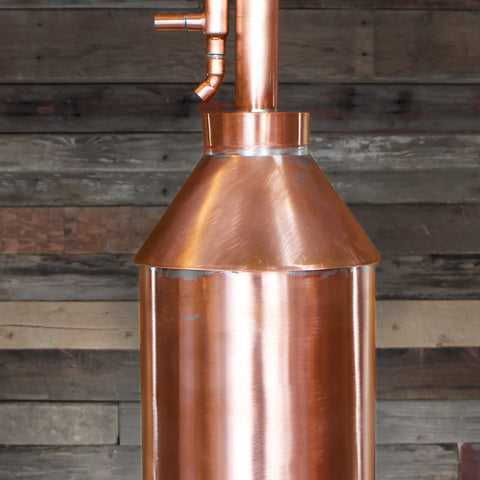This image showcases a shiny copper apparatus, resembling a still used in distillation, situated in a rustic wooden setting. The cylindrical copper machine, capped with a circular, hat-like top, features a series of curved and segmented tubes and pipes. These pipes extend from the main cylinder and appear to be disconnected from any external equipment. The detailed construction and gleaming surface of the copper appliance stand out against the backdrop of a log cabin wall, composed of various shades and textures of wooden planks. This scene evokes a sense of vintage craftsmanship and natural simplicity, highlighting the polished machinery against the earthy tones of the wooden wall.